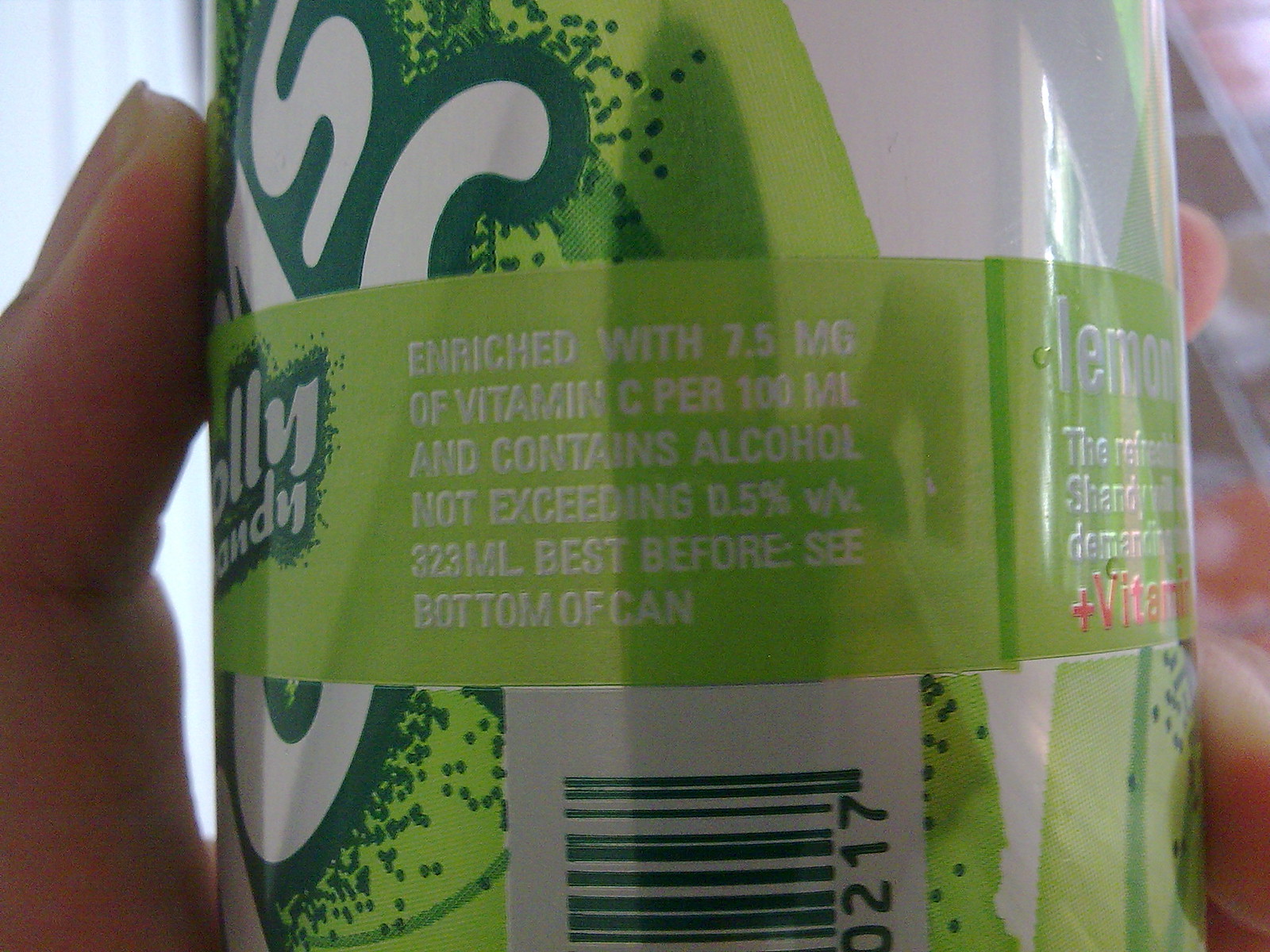The image is an up-close shot of a predominantly white and green soda can, held by a person's hand, with their thumb visible on the left and fingers on the right, although they appear somewhat blurry. The can bears the letters "O-L-L-Y" and "A-N-D-Y" on the left side, outlined in dark green letters. The majority of the can's surface is a light green, accented by a darker green in some areas, particularly in the outlines of the text. Around the center of the can is a light green stripe with text that reads: "enriched with 7.5mg of vitamin C per 100ml and contains alcohol, not exceeding 0.5% V/V, 323ml, best before C bottom of can." The bottom part of the can reveals a partially visible barcode. On the right side, the can features the word "lemon" prominently with further text that is mostly cut off due to the curve of the can, except for the words "this refreshing [...] shandy [...] plus vitamin." Hints of a QR code are also seen in the center section. The background of the image transitions from a light blue on the left side to a blurry surface, possibly the ground, on the right.